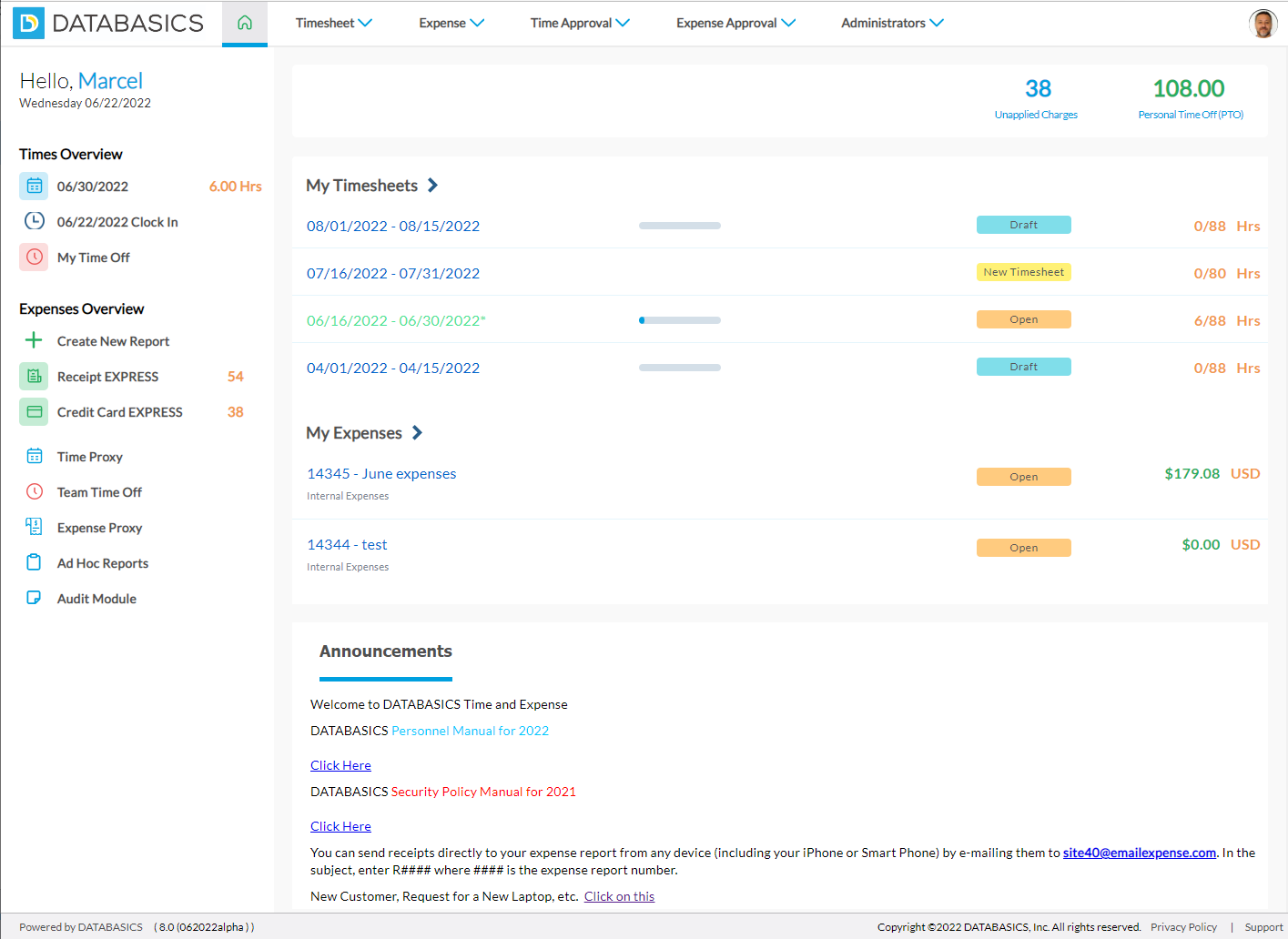The image displays a screenshot of a website with a predominantly white background. On the left side, there is a small blue square featuring a capital letter "D" in white. Adjacent to this square, the text "Databasics" is written in black, all as a single word. Below this logo, a gray square contains a green house icon with a blue underline at the bottom.

Further down the left side, the website greets the user with "Hello Marcel" where "Marcel" is in blue text. It indicates the date as Wednesday, 06/22/2022. The section is labeled "Times Overview" and lists entries such as "06/30/2022, 6 hours" and "06/22/2022 clock in." Additional options include "My Time Off," "Expenses Overview," "Create and Report," "Receipt Express," "Credit Card Express," "Time Proxy," "Team Time Off," "Expense Proxy," "Ad Hoc Reports," and "Audit Module."

At the top of the page, a banner displays tabs labeled "Timesheet," "Expense," "Time Approval," "Expense Approval," and "Administrators" along with a dropdown menu. On the far right of the banner, there is a small circular image of the user's face.

Below this banner, various sections are visible including "My Timesheets," "My Expenses," and "Announcements." The entries include status indicators such as "Draft," "New Timesheet," "Open," and "Zero Hours." The expense section shows detailed summaries of expenses.